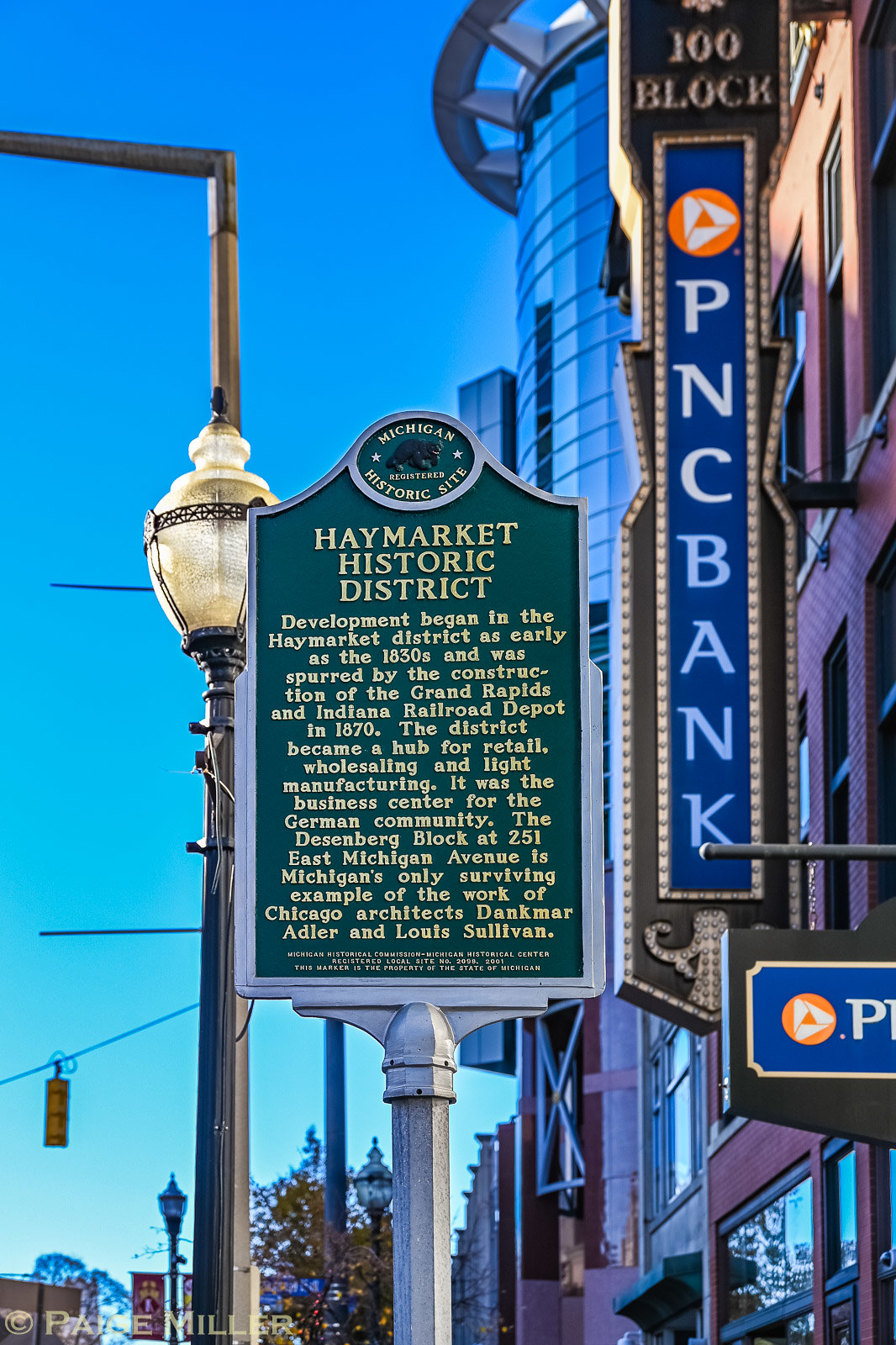This vibrant color photograph captures the essence of a historic downtown area under a clear, cloudless blue sky. The main focus is on an intricately designed green metal street marker mounted on an antique-looking post with gold lettering, proudly stating "Michigan Historic Site, Haymarket Historic District." The marker provides a detailed narrative, stating that development in the Haymarket District began as early as the 1830s, catalyzed by the construction of the Grand Rapids and Indiana Railroad Depot in 1870. It highlights the district's evolution into a hub for retail, wholesaling, and light manufacturing, and recognizes its significance as the business center for the German community. Noteworthy is the Dessenberg Block at 251 East Michigan Avenue, Michigan's sole surviving example of the architectural genius of Dankmar Adler and Louis Sullivan.

The scene is enriched by the surrounding urban landscape, featuring a charming, old-fashioned street lamp and multiple streetlights scattered across the area. A PNC bank is visible behind the historic sign, positioning itself as a backdrop to this quaint historic moment. The photograph's angled perspective offers a pleasant upward view, further emphasizing the pristine blue sky. Additional elements include some trees and other large buildings, contributing to the authentic downtown atmosphere. In the lower left corner, the copyright "Paige Miller" is subtly noticeable.